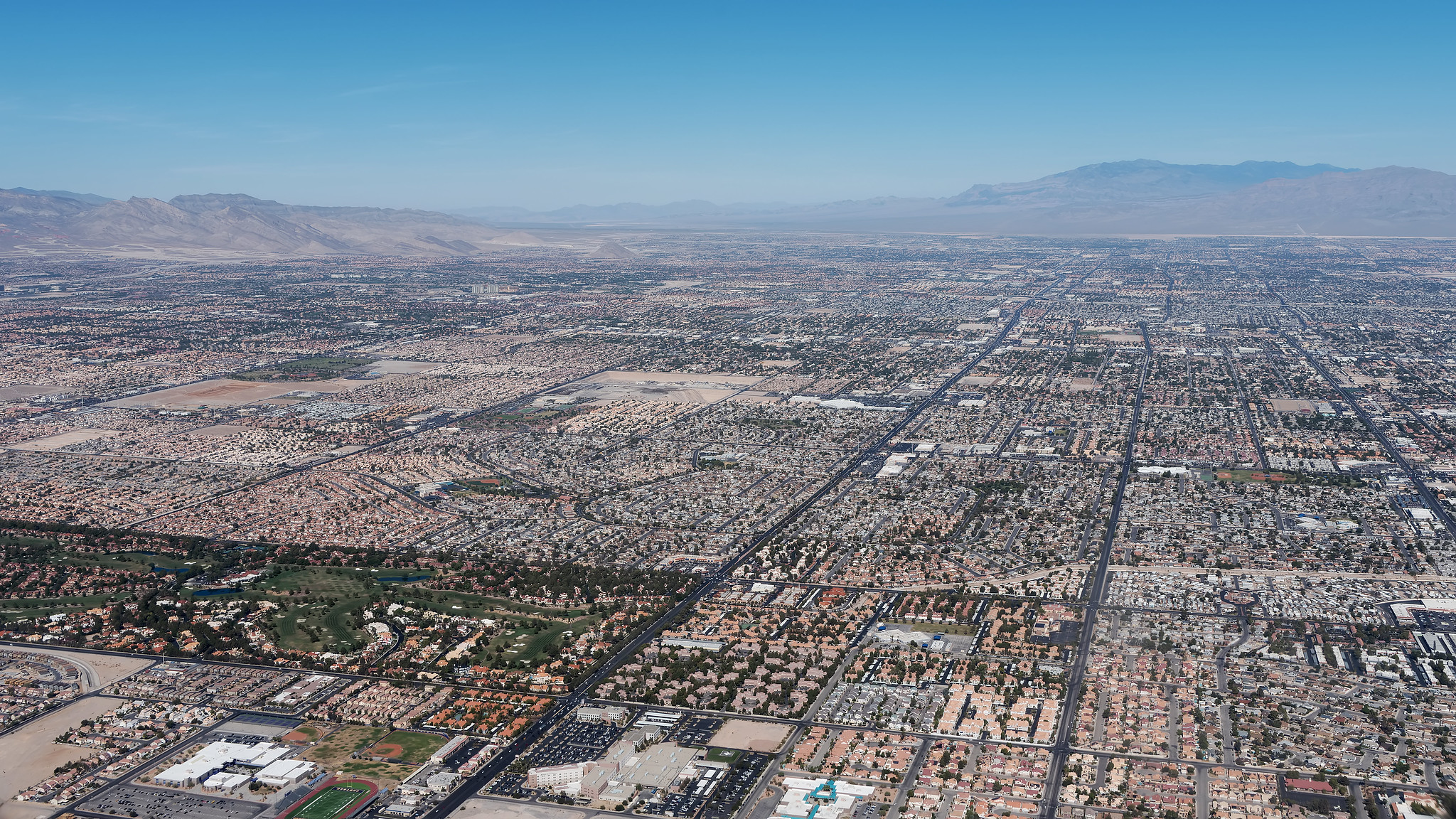In this breathtaking aerial photograph, a sprawling cityscape unfolds beneath a clear blue sky. The vast terrain is dotted with numerous neighborhoods, each distinguished by a patchwork of rooftops in varying hues of orange, brown, and white. Winding roads intricately weave through the communities, connecting the multitude of homes. In the distance, the city blends seamlessly into a landscape of rolling hills and valleys, creating a picturesque horizon where the vibrant terrestrial expanse meets the serene sky. This dynamic blend of urban intricacy and natural beauty captures the immense scale and vibrant diversity of a thriving metropolitan area.